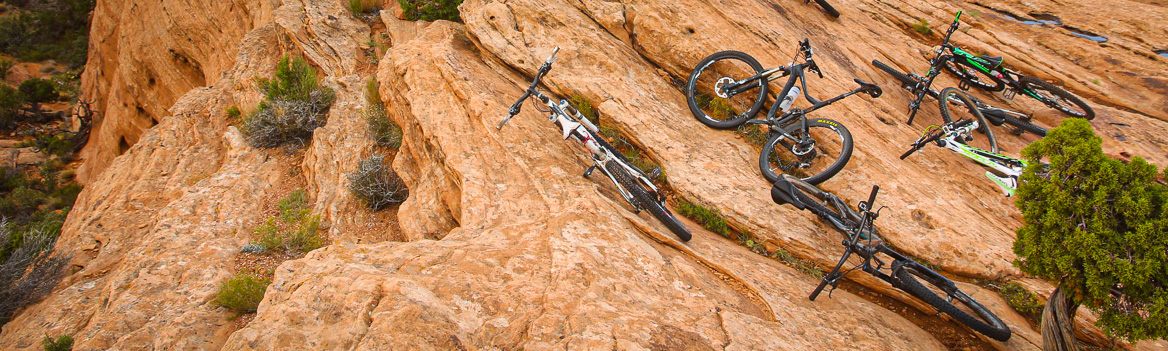This photograph captures a rugged canyon landscape adorned with an array of unmanned mountain bikes. The scene features a steeply angled, layered rocky cliff with tan and light brown hues, sloping at approximately a 40-degree angle. The rocky terrain is interspersed with several green shrubs and small trees, particularly noticeable in the crevices and towards the back right-hand corner. Here, a twisted plant with lush green foliage stands out prominently. The mountain bikes, predominantly black with some white and green details, are positioned on their sides across the rocky surfaces, highlighting the adventurous spirit of the terrain.